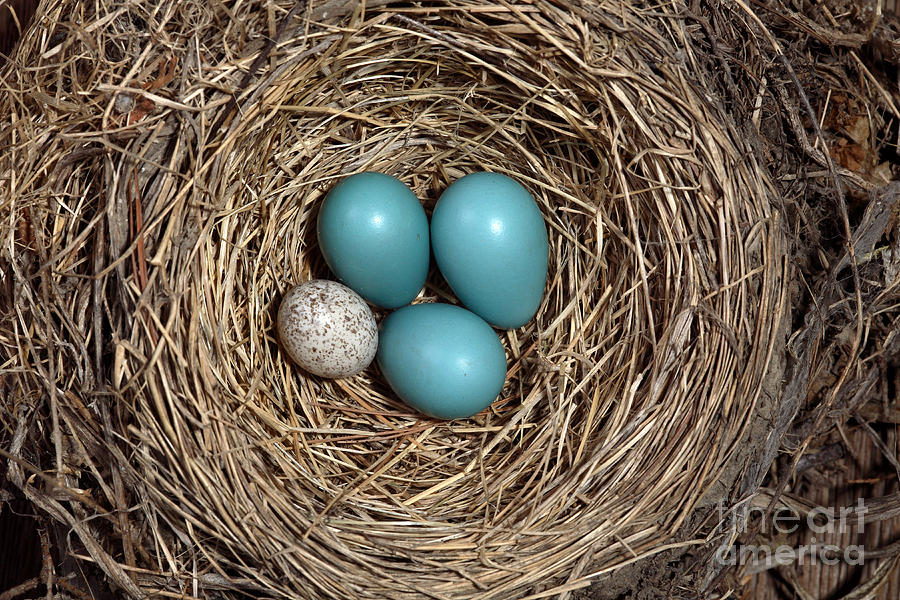This overhead landscape photograph showcases a bird's nest centered in the frame, occupying the entire vertical space and most of the horizontal space. The nest, constructed from an intricate arrangement of circular sticks and twigs in varying shades of brown, creates a thick, textured appearance. Only narrow slivers of the background are visible in the upper left and lower left corners, with a slightly larger portion of the background—comprising more sticks and natural debris—visible on the right side of the image.

At the heart of the nest lie four eggs. Three of them, resembling standard supermarket eggs in size, appear to be painted a light teal blue, reflecting light subtly. These three eggs are positioned almost in two rows: two at the top, closely aligned, and one directly below them. The fourth egg, noticeably smaller at approximately 60% the size of the others, is situated in the lower left of the nest. This smaller egg is white with brown speckles scattered across its surface.

In the bottom right corner of the photograph, a faded white watermark reads "Fine Art America," adding a professional touch to the image.